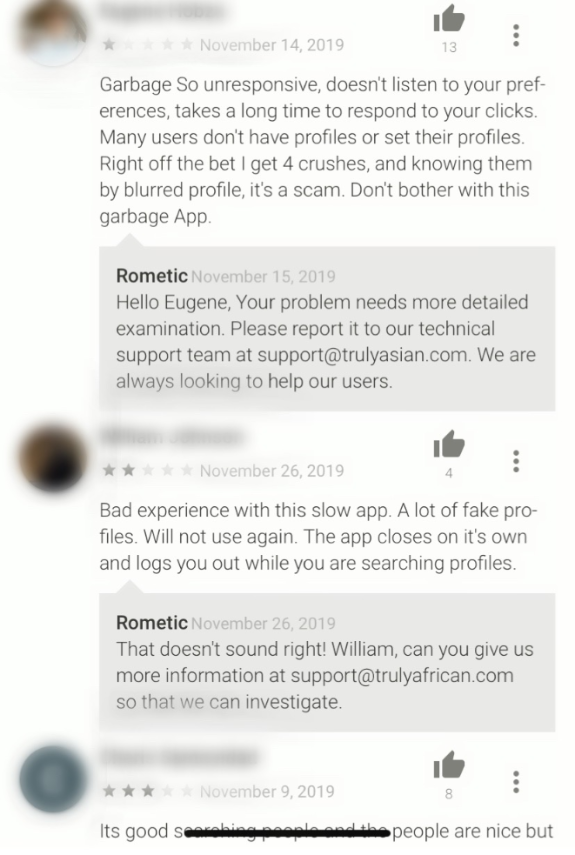**Screenshot of App Reviews with Responses**

This screenshot captures a series of reviews for an app, with the identities and icons of the reviewers obscured for privacy. 

At the top, a one-star review dated November 14, 2019, has received 13 thumbs up. The reviewer criticizes the app as "garbage," citing issues such as unresponsiveness, failure to adhere to user preferences, and slow responses to user clicks. They also mention that many users lack profiles or have incomplete profiles, leading them to suspect the app is a scam due to receiving four "crushes" from blurred profiles immediately. The app's representative, RoMedic, responded to this review on November 15, 2019, urging the reviewer to contact their technical support team for a more detailed examination of the problem. The response is highlighted in gray and emphasizes a commitment to user assistance.

The middle review, dated November 26, 2019, grants the app two stars and has garnered four thumbs up. This reviewer also reports a poor experience characterized by a slow interface, numerous fake profiles, and the app's tendency to close and log them out unexpectedly. RoMedic responded on the same day, expressing concern and asking for further details via their support email to carry out an investigation.

The final review, dated November 9, 2019, awards three stars and has eight thumbs up. However, only the first partial sentence of this review is visible, with the rest obscured by black ink.

Overall, the reviews reflect significant user dissatisfaction, with problems ranging from app performance issues to concerns about fake profiles. The app’s customer support team appears responsive, seeking more information to address the users' concerns.